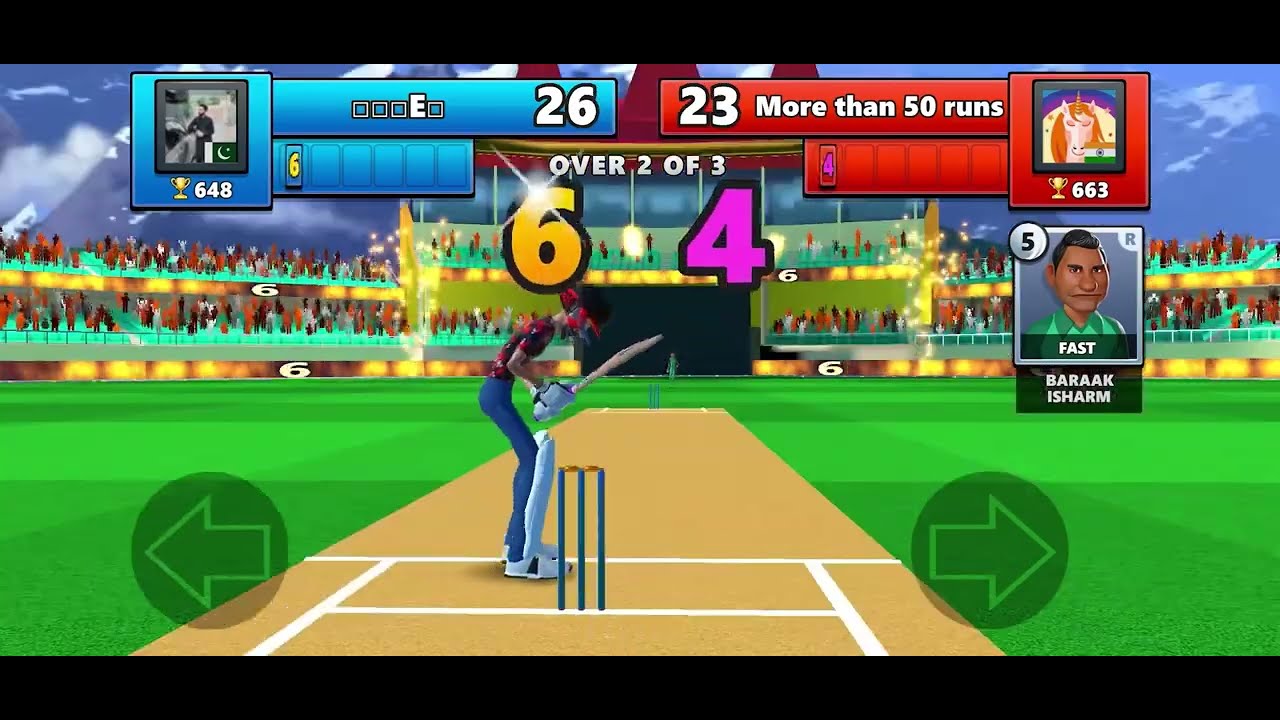The image is a screenshot from a video game that depicts a sports event, possibly resembling cricket or a similar sport. The central character, likely a robotic figure, is positioned in the middle of the screen holding an object that resembles a bat or sword. The figure is standing on a tan dirt pitch outlined with white lines, which runs centrally through the image. On either side of this dirt area is green grassy terrain. 

In the background, pixelated characters are seated as if they are spectators in a stadium, watching the event. The far background features mountains, adding depth to the scene. At the top of the screen, there are score sections for two teams: the blue team on the left, with a score of 26, and the red team on the right, with a score of 23, along with "more than 50 runs" noted. Both teams have trophy icons; the blue team shows a score of 648 while the red team displays 663. Below the red team’s score, there is an icon for a character named Barack Ishram, who is dressed in a green shirt and rated as "5R" with a descriptor "fast."

Annotations on the screen also include left and right arrow emblems to the right of the pitch, and notices like "over two of three" and the numbers six and four highlighted in orange and pink respectively.